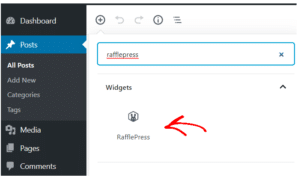This image is a blurry, low-resolution screenshot set against a white background. At the top of the image, there is a dark gray line spanning across. On the left side, there is a vertical navigation bar with a black background, displaying various menu options in white text. The topmost option is "Dashboard," accompanied by an icon. Below it, highlighted in blue, is "Posts" with a pushpin icon. Further down, in sequence against the black background, are "All Posts," "Add New," "Categories," "Tags," "Media," "Pages," and "Comments."

To the right part of the image, against the white background, a blue-outlined white box appears with the text "RafflePress" underlined in red. Below this, in dark gray print, the word "Widgets" is visible, along with a red left-pointing arrow labeled "RafflePress." Additionally, there is a small icon resembling a bunny rabbit's head situated near the "RafflePress" label.